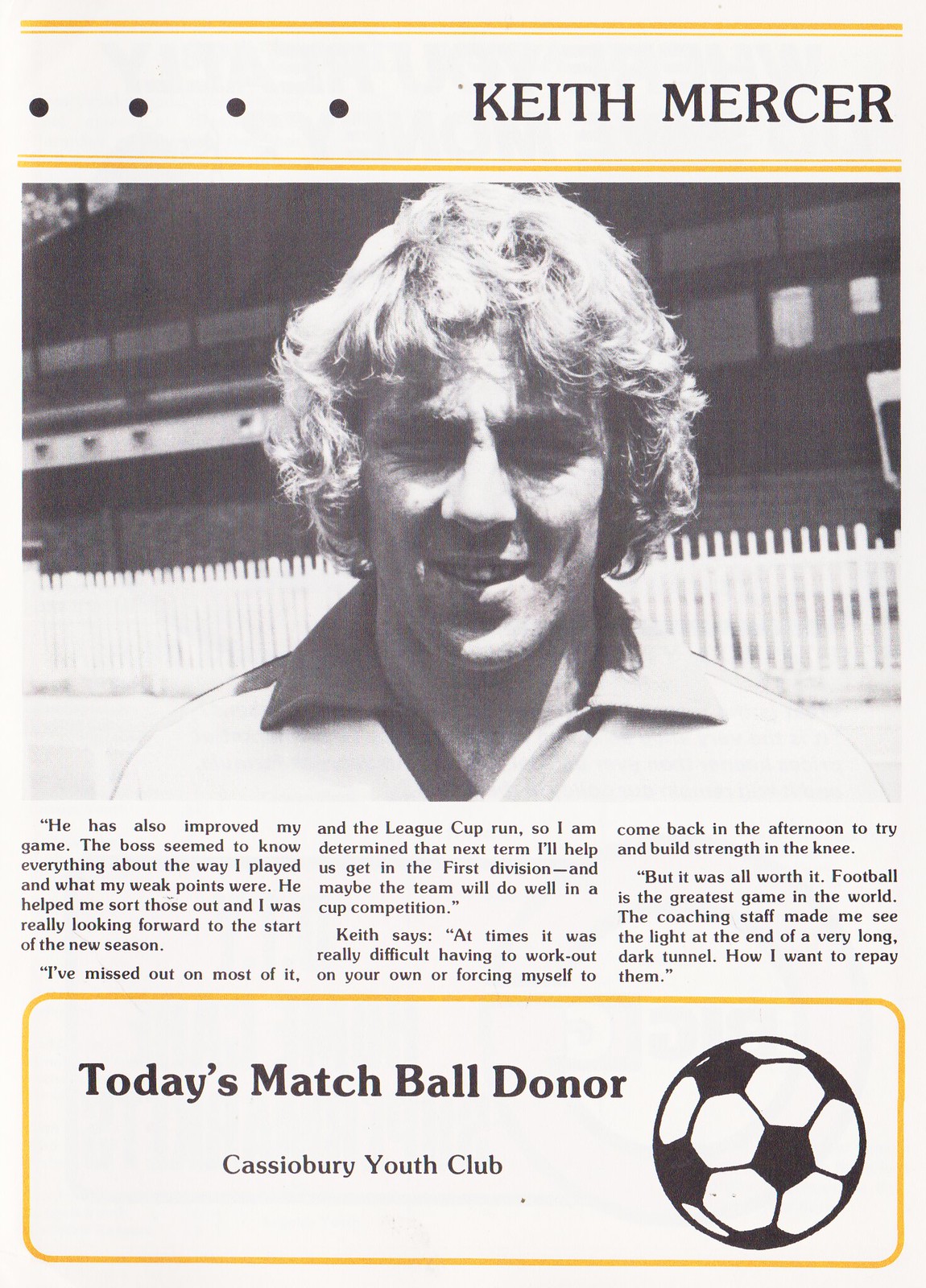This image is a vertically aligned rectangular clipping that appears to be a faded page from an old newspaper or magazine. The page features a detailed article about a player named Keith Mercer. The background is white, and the top of the page is bordered by two horizontal yellow lines with some colored circles on the left side. Between these lines, in all-caps black text, it reads "KEITH MERCER." Below the heading, there is a black and white photograph of Keith Mercer, who is smiling at the camera. He has shaggy, wavy hair that falls over his ears and is wearing a collared shirt, standing outdoors in front of a large building and a white picket fence.

Beneath the photo, there are three short columns of text summarizing Mercer's thoughts and experiences. He discusses how his coach helped him improve his play by addressing his weak points, his determination to perform well in the upcoming season, and his challenges in recovering from a knee injury. At the bottom of the clipping, framed by a rounded yellow rectangle, the caption states: "Today's Match Ball Donor: Cassiobury Youth Club," accompanied by a black and white image of a soccer ball on the right side.